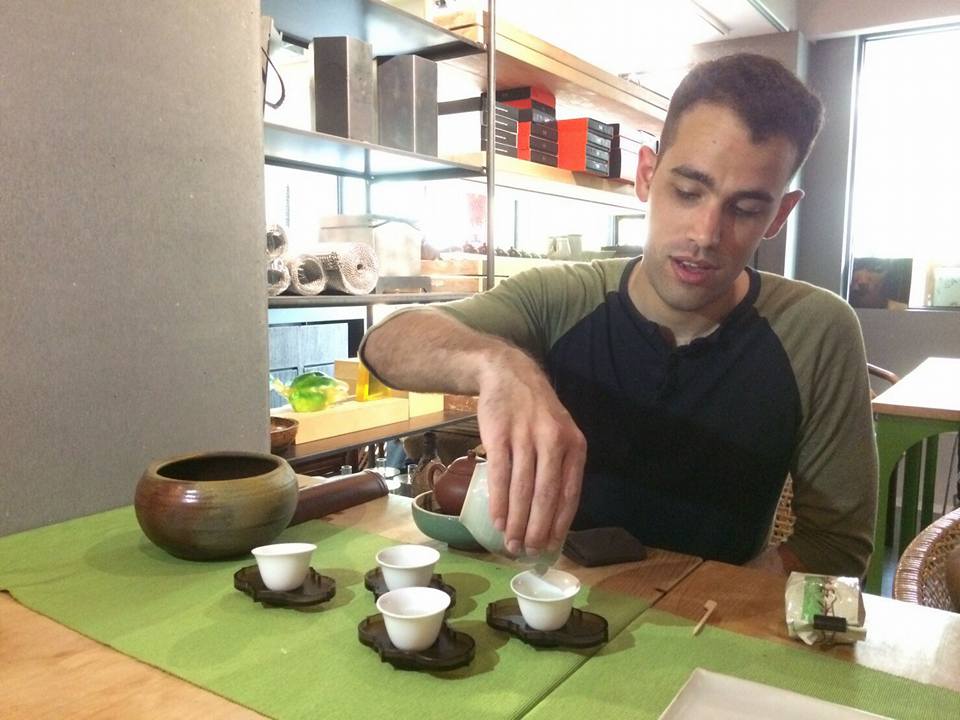In this image, a young man with brown skin and a distinctive V-shaped hairstyle sits at a wooden table adorned with a pea green table runner, situated in a brightly lit commercial kitchen or restaurant. He wears a long-sleeve, two-tone green and black jersey-style shirt, with sleeves rolled up to his elbows. In front of him are four white porcelain teacups, each nested on little trays, and he is seen carefully pouring a liquid from a celadon green jug into the teacups. Additionally, a terracotta-colored teapot is placed in a ceramic bowl on the table, alongside a bag of matcha green tea and a traditional wooden whisk used in Japanese tea ceremonies. The background reveals stainless steel shelving holding various kitchen items, and natural light streams in from a window, illuminating additional tables and chairs in the restaurant setting.